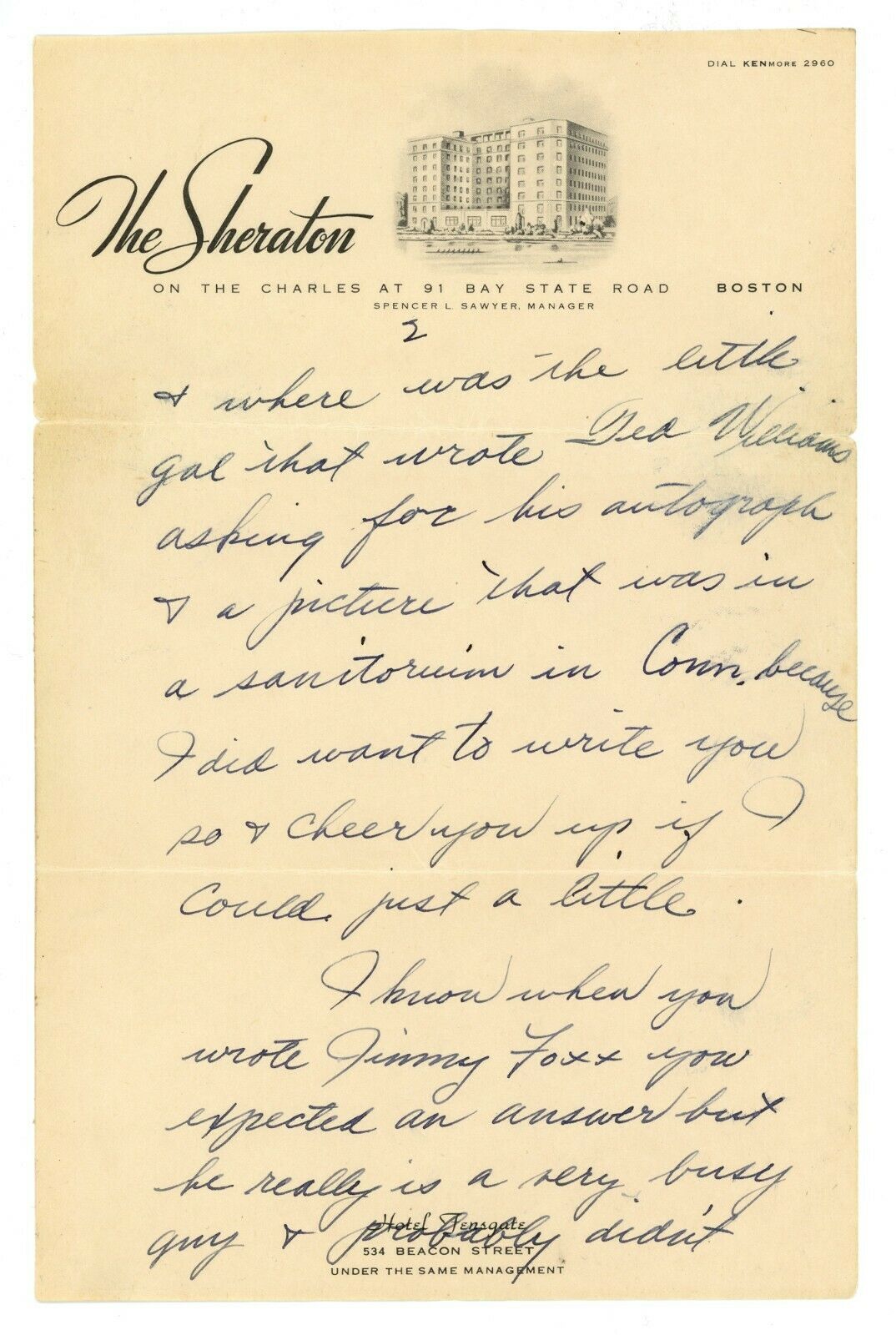The image shows an old, vintage letter on discolored, peach-colored notepaper from the Sheraton at 91 Bay State Road, Boston. The upper left-hand corner features a detailed black and white illustration of the Sheraton Hotel, labeled "Sheraton on the Charles," with the address and the manager’s name, Spencer L. Sawyer, written nearby. In the upper right-hand corner, there is a note in black font saying "Dial Kenmore 2960." Below these details lies a handwritten note in black cursive ink, spanning about two paragraphs, though parts of it are illegible. The note seems personal and mentions someone asking for an autograph and a picture, as well as references to Jimmy Fox. At the very bottom, beneath the cursive writing, the text reads "Hotel Gensate, 534 Beacon Street, under the same management." This intricate letter combines elements of formal hotel stationery with a personal, heartfelt message.